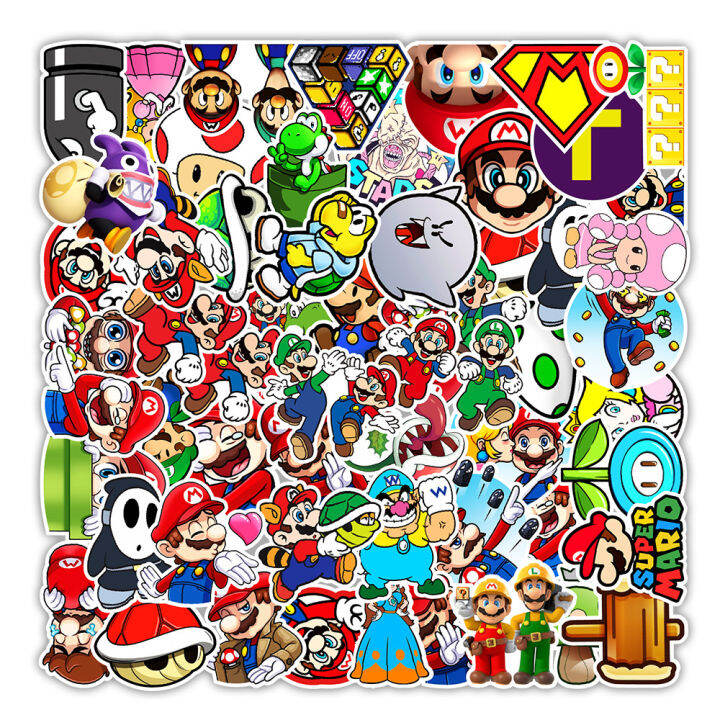This square frame illustration is a vibrant and chaotic collage brimming with countless small, compact logos and sticker-like illustrations from the Mario Brothers franchise. Set against a scarcely visible white background, hundreds of overlapping images, mostly round-shaped, create a dazzling, colorful tapestry. Predominantly featuring Mario in various poses and facial expressions—over twenty in total—the collage also showcases a plethora of other iconic characters such as the Mushroom character, Princess Peach, and game elements like question mark cubes, gavels, ladders, and an 'M' shaped Superman logo symbolizing Mario. The entire composition is packed densely with vivid cartoon colors, leaving no space unfilled.